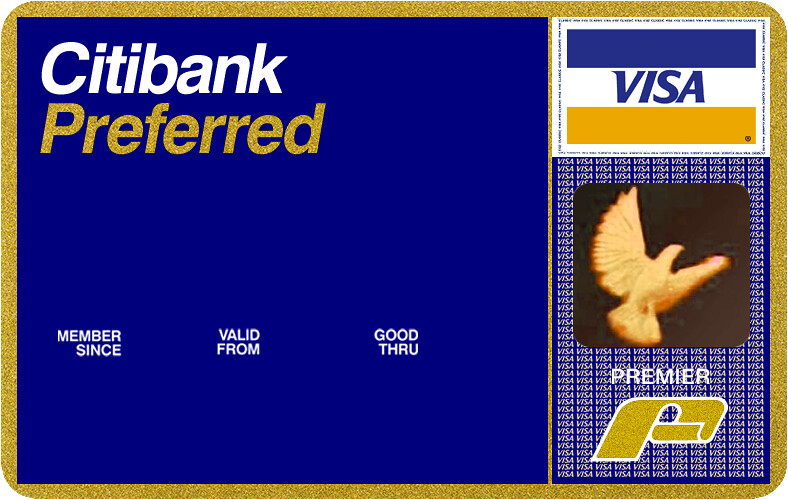This is an image of a Citibank Preferred Visa Premier card, presented without any identifying information, likely for demonstrative purposes. The card itself is predominantly royal blue with a gold glittery rim around its perimeter. In the upper left-hand corner, the text "Citibank" is written in a white, slightly italicized sans serif font, followed by the word "Preferred" in a gold, similarly italicized font. Along the lower left section of the card, placeholders for "Member Since," "Valid From," and "Good Through" are marked but left blank. 

In the upper right corner, the Visa logo is prominently displayed, characterized by a design resembling a flag with a navy blue stripe on top, a white middle, and a mustard yellow bottom stripe, with the word "Visa" in navy blue font centered on the white stripe. Below the Visa logo, there is a hologram of a flying bird, likely a pigeon or dove. At the bottom right section, the word "Premier" is denoted below the card logo, featuring a gold and white letter "P." The overall design emphasizes a sophisticated blue and gold color scheme, with clean lines and a focus on branding elements.